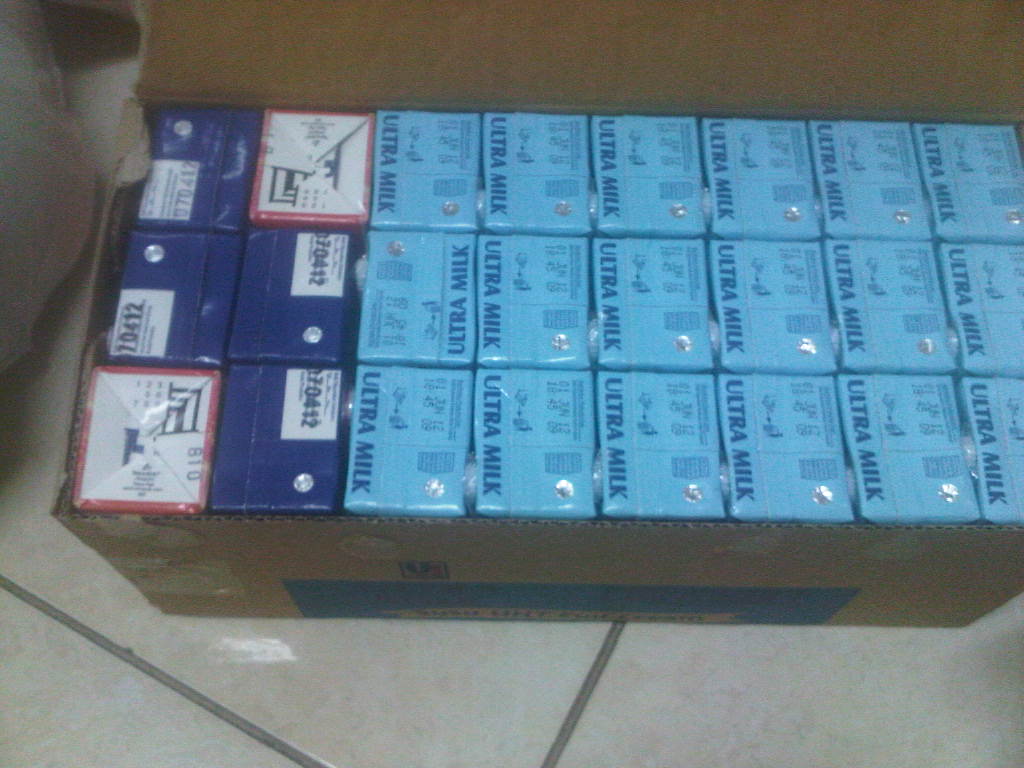The close-up, slightly fuzzy photograph in color captures an open brown cardboard box containing multiple milk cartons, prominently placed on a white tile floor with dark gray grouting. The flaps of the box are pushed to the right, revealing its contents. The box has a blue rectangle on its side, the text on which is unreadable due to the angle and quality of the image. Inside, there are different types of milk cartons: Four dark blue cartons with numbers "70412" on the tops, and two of these are flipped to display their bottoms with "810" marked in dark blue, encircled by red lines and white spaces. In addition, partially visible light blue cartons labeled "Ultra Milk," featuring a small silver circle for the straw, are present on the right. The cardboard box is located adjacent to the edge of a fabric piece, contributing to the overall composition of this detailed and descriptive scene focused on milk storage in a domestic setting.